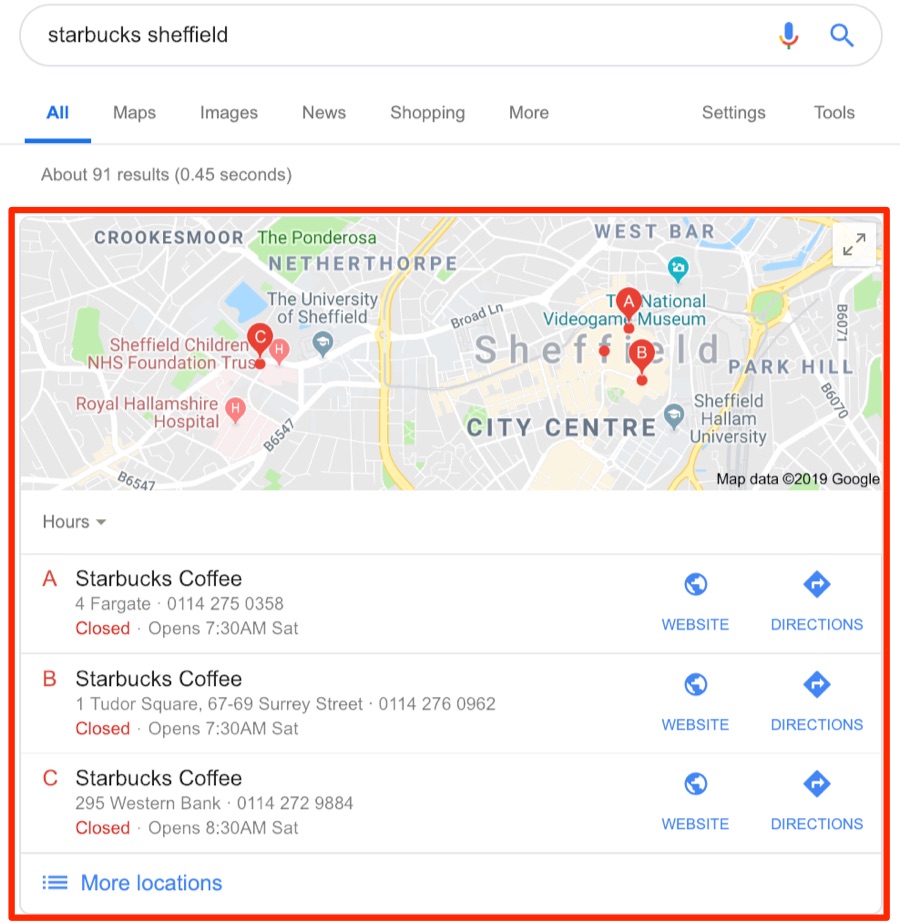A screenshot of a search results page for "Starbucks shops in Sheffield" is displayed. At the top, various tabs are shown: All, Maps, Images, News, Shopping, More, Settings, and Tools. Additionally, it states "About 91 results" in grey text. The image features a red-outlined box highlighting the Sheffield area, with three labelled points: A, B, and C, each marking a Starbucks location.

- **Point A: Starbucks on Fargate**  
  Situated close to downtown Sheffield, this Starbucks is currently closed but will reopen at 7:30 a.m. on Saturday. The website and directions are available in blue hyperlinks.

- **Point B: Starbucks on Tudor Square**  
  Located slightly south of Point A, at 67-69 Surrey Street, this Starbucks shares the same opening hours as Point A, reopening at 7:30 a.m. on Saturday. Similarly, its website and directions are accessible via blue hyperlinks.

- **Point C: Starbucks near the Sheffield Children's NHS Foundation Trust**  
  This Starbucks, located on Western Bank, is further away from the city center compared to Points A and B. It remains closed and is scheduled to reopen at 8:30 a.m. on Saturday, with the website and directions similarly highlighted in blue.

Beneath Point C, there's additional text reading "More locations," also in blue, indicating further Starbucks locations in the area.